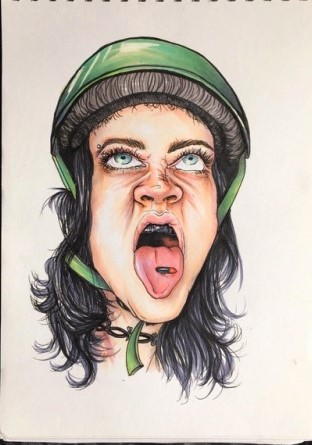The image features a seemingly discontented teenager, identified as likely being female, with her mouth wide open as if in a scream or rant. She has long, wavy black hair and blue eyes accentuated by long, possibly made-up lashes. The teenager is wearing a green helmet with a grey lining, and green straps fastened under her chin. Around her neck is a black chain. Her tongue, which is noticeably large, has piercings. Her teeth are visible and appear discolored, almost black. The girl's facial expression is contorted as she looks upwards. In the background, there are indistinct red and black blobs.